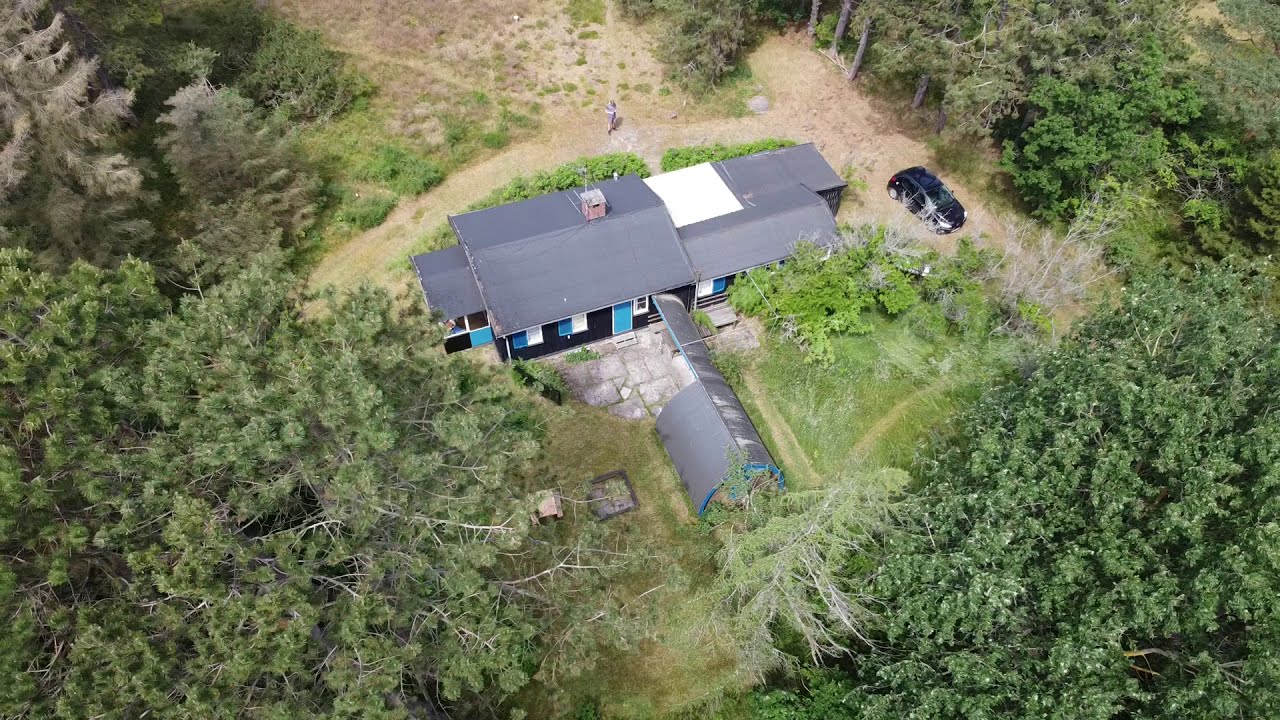An aerial view showcases a single-story house painted black with teal trim and a gray roof, situated at the center of the image. The house, which exudes an eco-friendly appeal and features blue doors and shutters, is set within a large clearing amidst dense, varied green pine trees and bushes. To the front of the house, slightly towards the bottom of the frame, there's a teal-colored shed or barn with a gray roof, and what appears to be a cylindrical structure, possibly a greenhouse. The property includes a dirt driveway extending to the left under a tree that dominates the lower left quadrant, while the lower right quadrant is filled with more trees. A black car is parked at the end of the driveway to the right of the house. Beyond a row of green hedges behind the house, there appears to be a person looking down at their camera, backdropped by a brown, weed-covered ground.